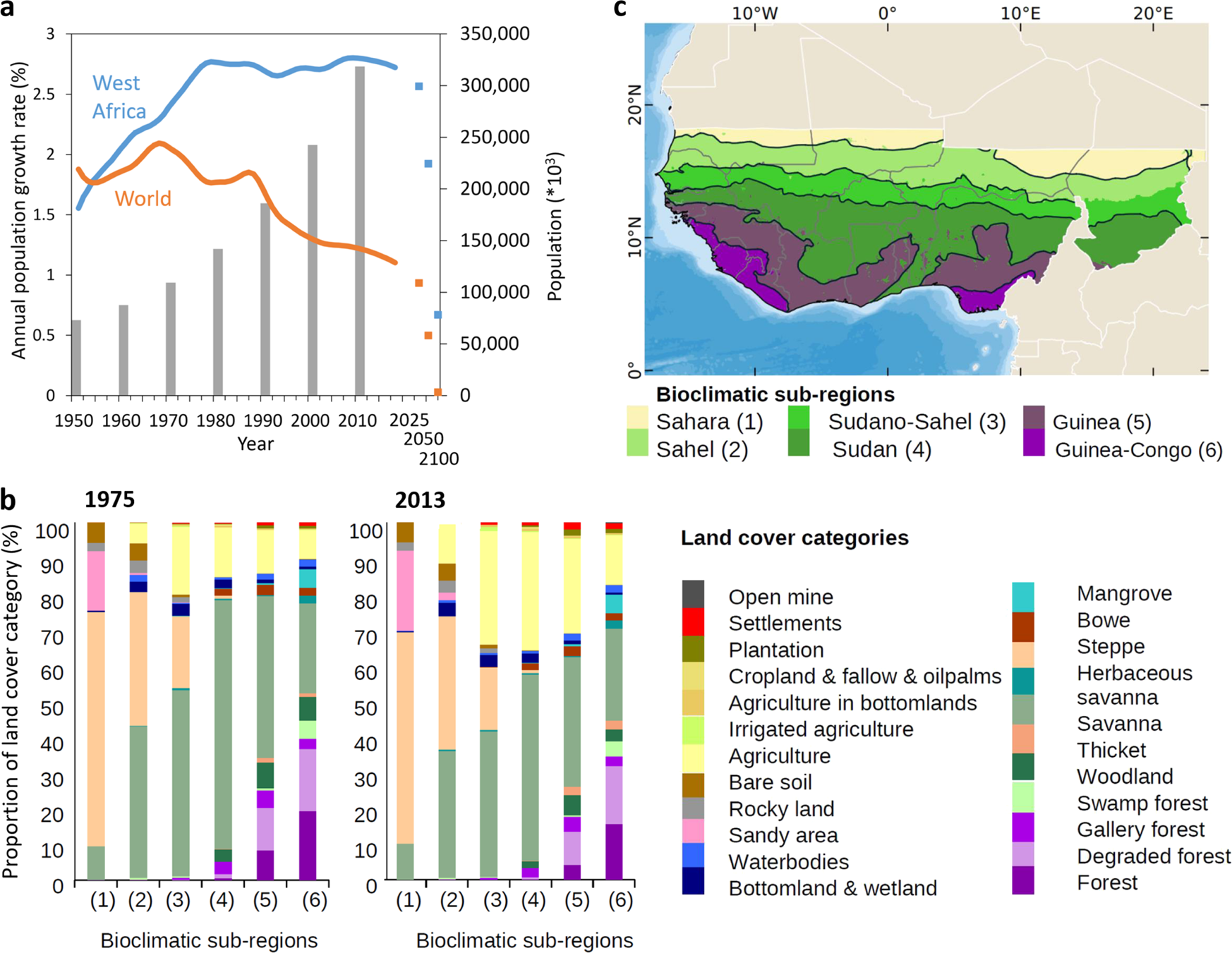The image showcases a detailed comparison of various environmental and demographic metrics. In the top left corner, Chart A illustrates the annual population growth rate from 1950 to projections in 2050. It features two distinct lines: a gradually declining orange line representing global trends and a steadily increasing light blue line indicating West African trends. To the bottom left, Chart B displays the proportion of land cover categories in bioclimatic sub-regions for the years 1975 and 2013, highlighting different land types such as open mines, settlements, plantations, cropland, and various natural landscapes. Bioclimatic sub-regions, including Sahara, Sahel, Sudano-Sahel, Sudan, Guinea, and Guinea-Congo, run along the x-axis. To the right, an accompanying map of West Africa vividly color-codes these bioclimatic sub-regions and detailed land cover categories, providing a comprehensive visual representation of the ecological makeup, including water bodies, wetlands, mangroves, savannas, forests, and rocky lands. The image effectively combines demographic and ecological data to give an in-depth look at West Africa's evolving landscape over time.